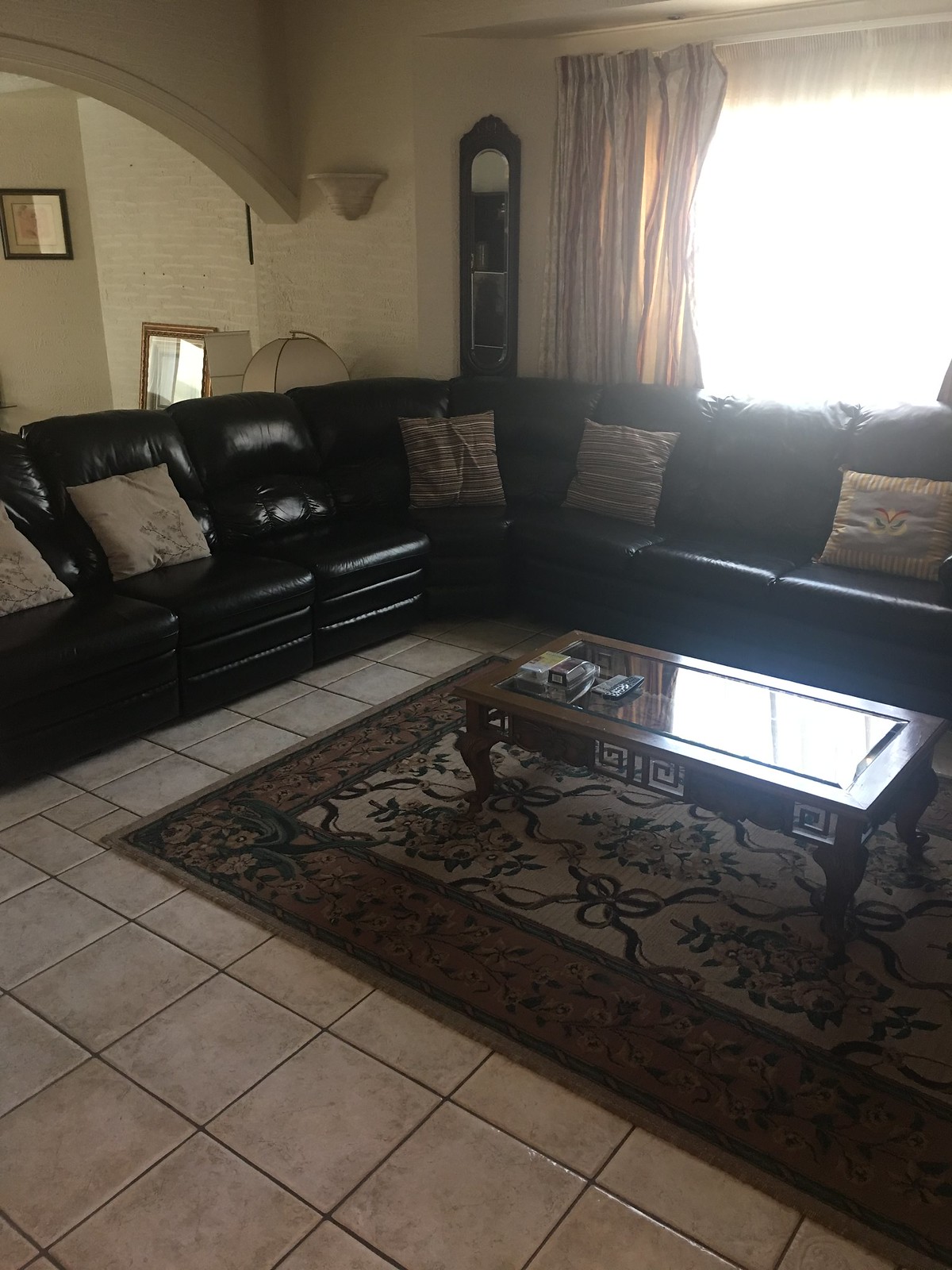This detailed photograph showcases a living room adorned with ceramic tile floors featuring black grout lines. The central area is anchored by an ornate, mosaic-style rug that incorporates off-white, floral center patterns and a brown border embellished with yellow flowers and a green outline. A glass-topped wooden coffee table with curved legs and intricate spiral designs occupies the center space, flanked by a large black leather sectional that can comfortably seat up to 12-14 people, adorned with brown and yellow throw pillows.

The backdrop includes white painted brick walls and a large picture window with tan, striped curtains that allow bright light to flood the room. An elegant standing clock is positioned behind the sectional, next to a rounded lampshade peeking out from the same area. Several wall ornaments, including placards and paintings, add a personal touch to the decor. A curved archway leads to another room, enhancing the open and spacious feel of this living area. Small items are subtly placed on the corner of the coffee table, adding to the lived-in charm of this cozy yet sophisticated space.